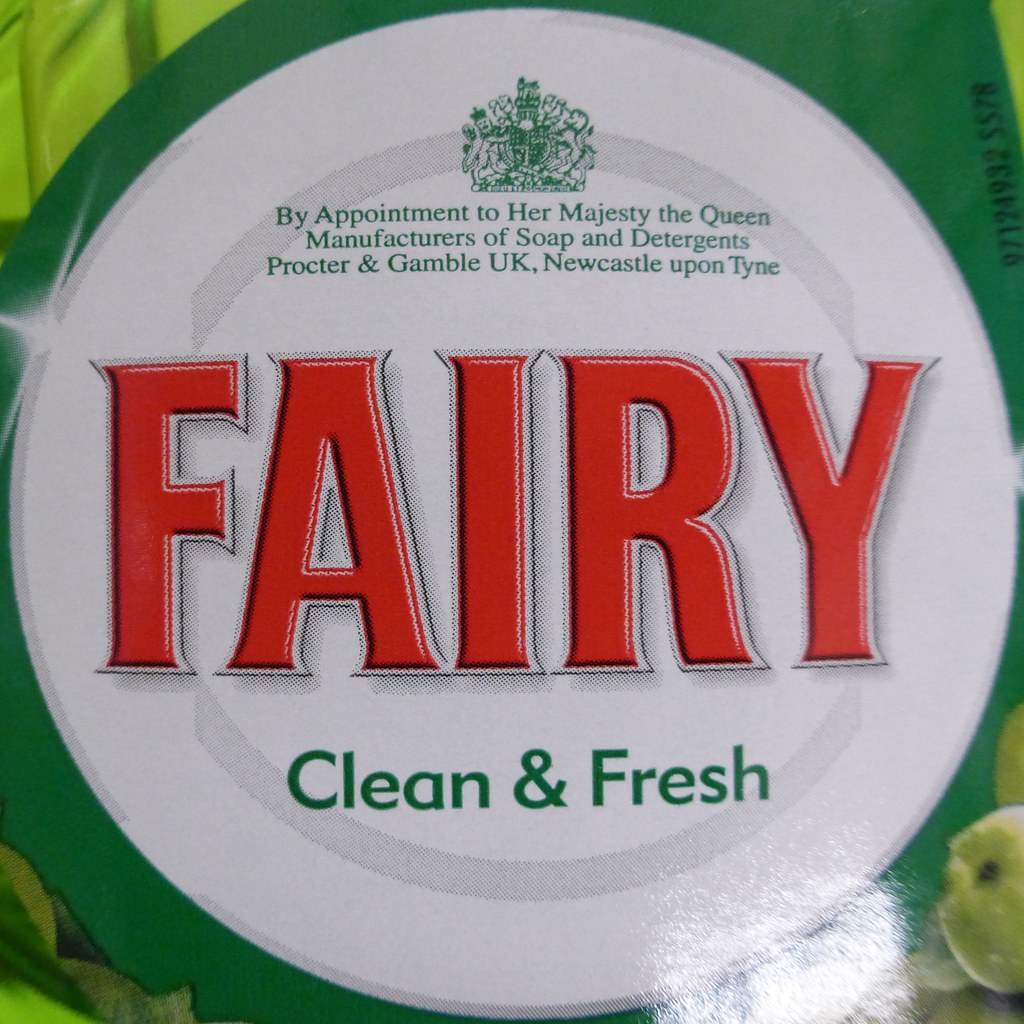This close-up photograph features the logo and branding of a household cleaning product, likely dishwashing soap or washing machine detergent, prominently displayed on its packaging. The central focus of the image is a circular logo with a white background. In the center of this circle, the word "FAIRY" is prominently written in large, bold red capital letters. Directly below, in smaller green capital letters, is the phrase "CLEAN & FRESH." Above "FAIRY," there is an intricate green emblem featuring two lions leaning against a throne topped with a crown. Surrounding this emblem is a text that reads, "By Appointment to Her Majesty The Queen Manufacturers of Soap & Detergents Procter & Gamble, UK, Newcastle upon Tyne." The circular logo is bordered by alternating areas of dark and light green. In the bottom right corner of the image, a green apple is visible, adding a touch of realism as some granular soap appears to have spilled nearby on the packaging. The background colors and detailed elements all contribute to the overall impression of the product being either in a store or in a household setting.